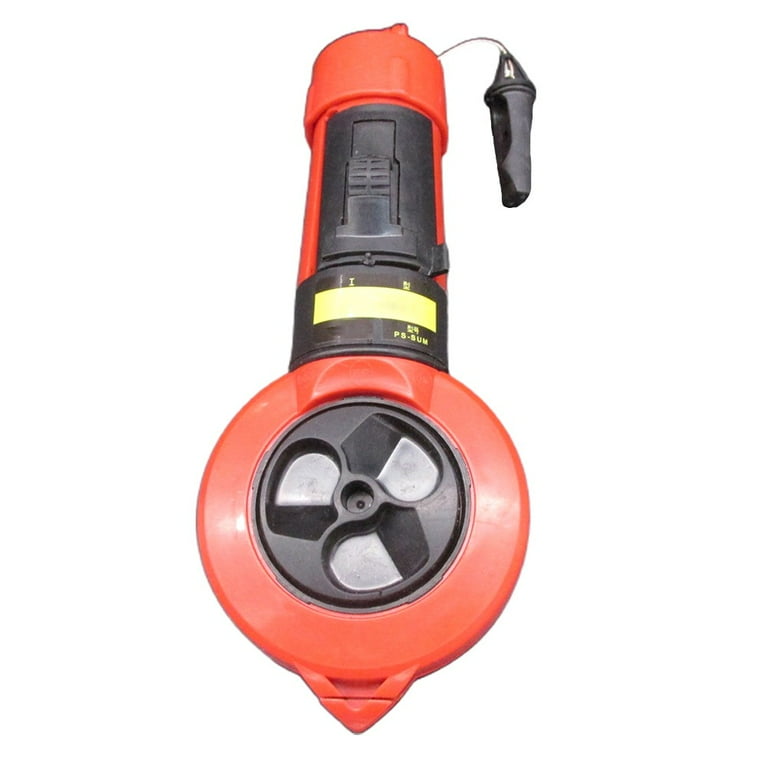This image is a detailed color photograph of a tool set against a plain white background. The central object resembles a hybrid between a flashlight and a handheld fan. It features an orange cylindrical body, with the lower part widening into a round, orange base that has a distinctly blunt, spiky triangular end. Above this, there's a round, black section housing a fan-like component with three silver blades, giving it an appearance akin to a hubcap.

Moving upwards, the midsection of the tool is black and serves as a handle, with a prominent yellow stripe running across it that possibly displays indistinct lettering or numbers, potentially reading "PS SUM" or "P5 SUM." This part also includes an on-and-off switch. Stemming from this black handle is a thin string attached to a black piece resembling a whistle.

On the side of this black section, a plastic whistle-like component, attached by a silver wire, extends outward. Overall, this tool seems multifunctional, incorporating elements of both a fan and a flashlight, with a design that suggests it might plug into a car dashboard or a cigarette lighter socket.